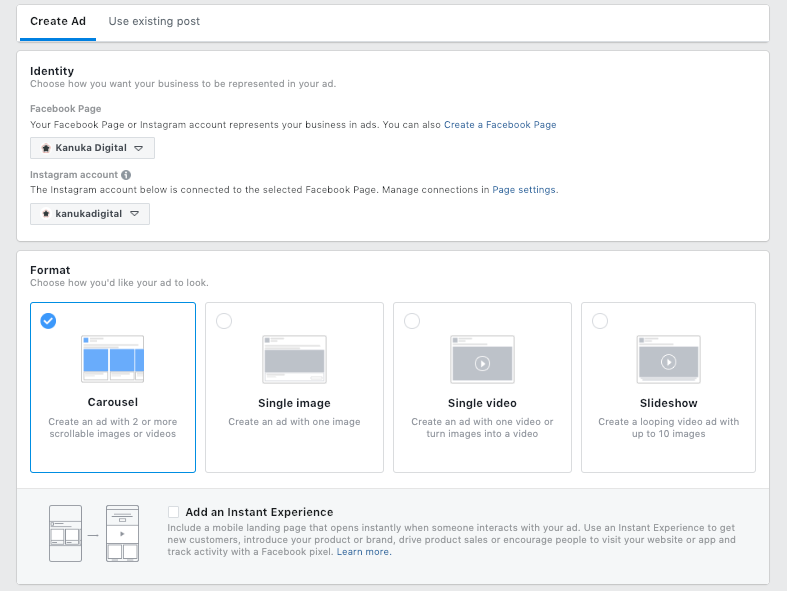The image displays a screenshot of an advertisement creation interface set against a light gray background with a white header at the top. On the upper left of the header, the text "Create Ad" is prominently underlined in blue, while to the right, "Use Existing Post" is displayed. 

Below the header, there's a white box titled "Identity." Inside this box, the text instructs, "Choose how you want your business to be represented in your ad." A button labeled "Canuca Digital" is available with a drop-down menu, representing options for selecting the business identity. Another identical button labeled "Canuca Digital" features a drop-down menu as well, intended for selecting either the relevant Facebook Page or Instagram account.

Further down, another white box is present, this time titled "Format" in bold black text. This section invites users to "Choose how you'd like your ad to look," offering four distinct format options, each illustrated with images. The first option on the left is "Carousel," allowing users to create an ad with two or more scrollable images or videos. The second option, "Single Image," is for creating an ad with one image. Next is "Single Video," which lets users create an ad with one video or turn images into a video. Lastly, the "Slideshow" option enables the creation of a looping video ad with up to 10 images.